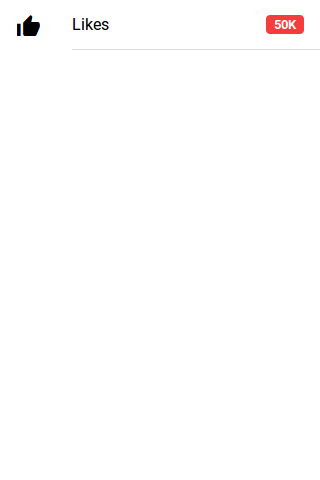The image features a clean white background with various black text elements. In the top left corner, there is a black thumbs-up icon, representing a "Like" button. To the immediate right of this icon, the word "Likes" is prominently displayed in black text.

In the top right corner, a red square with rounded corners stands out. Inside this square, the number "50k" is displayed in white, indicating the quantity of likes. Beneath the word "Likes" and the "50k" label, there is a thin, gray horizontal line that separates these elements, adding a touch of subtlety to the design.

The overall message of the image is to provide feedback on a certain piece of content, such as a video or post, highlighting that it has received 50,000 likes. The visual emphasis on the thumbs-up icon and the prominent display of the number 50k reinforces the popularity and approval of the content among viewers.